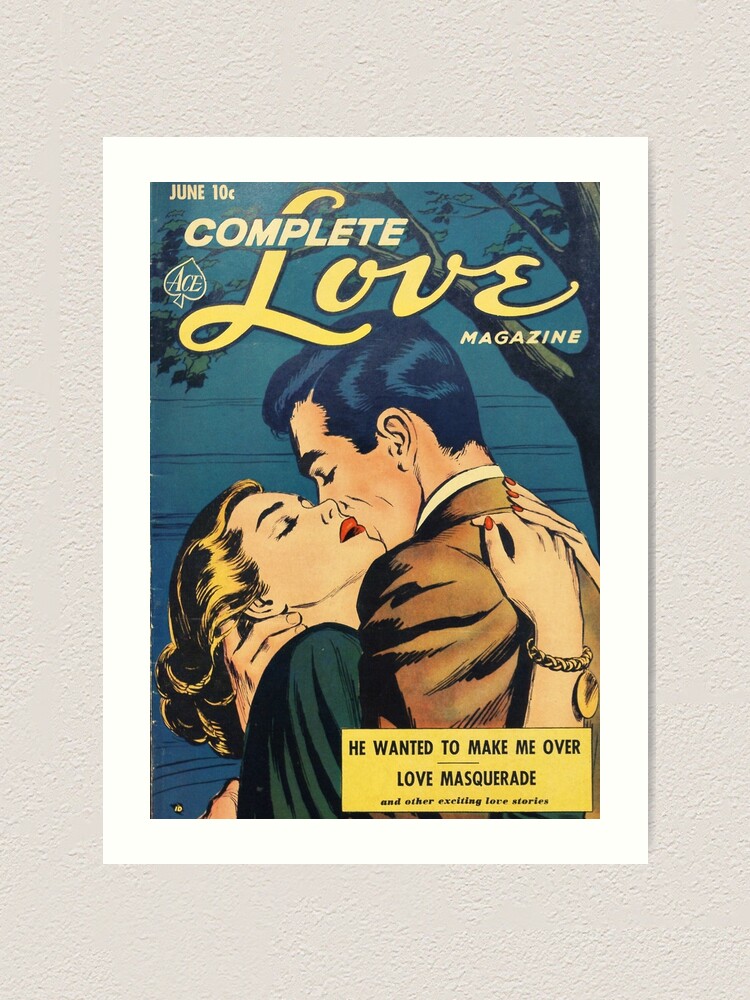The cover of the vintage comic-book style Complete Love Magazine, priced at 10 cents and issued in June, features an intimate, close-up drawing of a man and woman embracing outdoors beneath a tree. The title "COMPLETE LOVE MAGAZINE" is prominently displayed, with "Complete" in bold capitals, "Love" in cursive, and "Magazine" again in capitals. The man, with closely cropped, coiffed dark hair, is dressed in a beige suit with a white shirt, while the woman, characterized by her golden, dark blonde hair and vivid cherry red lipstick, is wearing a green outfit and a charm bracelet on her right arm. Her neck is slightly arched back as she receives a near-mouth kiss from the man. The bottom right of the cover features the phrases "He Wanted to Make Me Over" and "Love Masquerade," hinting at the exciting love stories within.